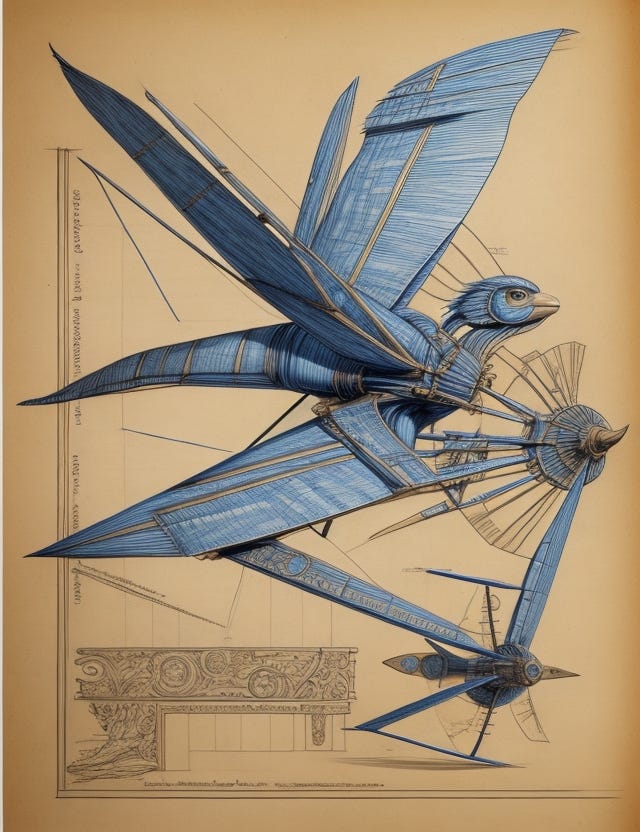The image is a highly detailed and stylized illustration, presenting a fusion between a bird and an airplane on an aged, yellowed backdrop. Dominating the illustration is a large, blue bird accented with gray and beige stripes, intricately displaying its anatomy in flight. The bird's beak and wings are meticulously taken apart and shown in segments, analogous to airplane components such as flaps and a propeller, unraveling the mechanics of its flight. The background features very fine, illegible print, contributing to the vintage aesthetic. At the lower left corner, there is a sketch in pencil, resembling an elaborate desk or a column-like structure. Additional elements include another bird-like creature at the bottom, standing with two wings atop a rod, and a bird's head detailed with a closed beak and an open eye, enhancing the illustration's blend of natural and mechanical motifs.